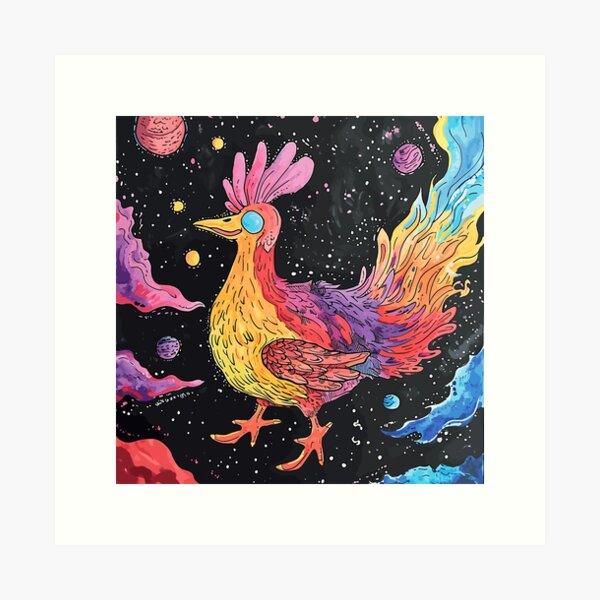This is a highly detailed, vibrant digital artwork entitled "Space Rooster." The overall piece is vertically rectangular and includes a very faint light blue or light gray outer border surrounding a white inner border; the main image itself is square. The background is the blackness of space dotted with numerous white stars, creating a cosmic canvas. Several multi-colored planets, including yellow, red, purple, and orange ones, float around the scene, along with colorful space dust and clouds in hues of purple, blue, and red.

Dominating the composition is a massive, fantastical rooster sailing through space. This "Space Rooster" has brilliantly colorful feathers with shades of yellow, red, purple, orange, and blue. A striking feature is its enormous, solid blue eyes and a red headpiece. The rooster's tail explodes into a spectacular display of multi-colored flames, primarily featuring red, orange, yellow, and blue. Its underbelly glows a bright yellow, while its feet are vividly red. The whole scene exudes a surreal, psychedelic vibe that is both enchanting and otherworldly.